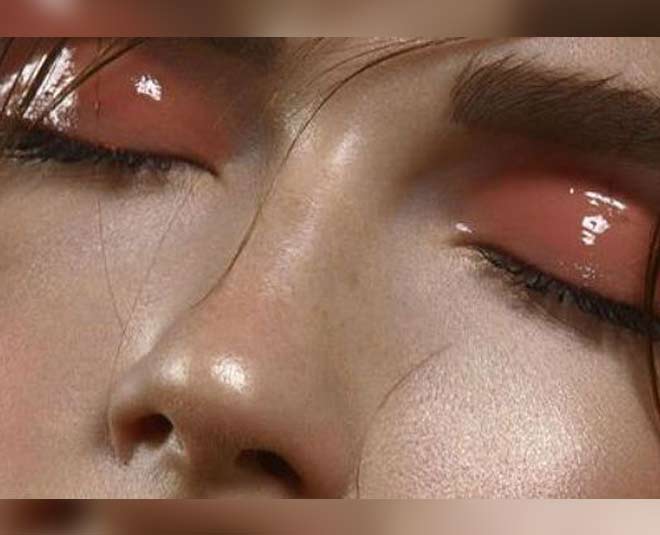This image is a detailed close-up of a woman's face, focusing primarily on her eyes, eyebrows, and nose. The photograph excludes her hair and only shows up to the bottom of her nose. Her head is tilted to the right side of the picture, and her eyes are closed, adorned with a glossy, pink eye shadow that gives a wet appearance with noticeable reflections on her eyelids. Her facial skin is pale and somewhat reflective, with brighter shines on the tip of her nose, her cheekbone, and the bridge of her nose. The woman's eyebrows are brown, with the left one partially cut off at the edge of the image. Strands of her brown hair drape slightly across her face. The overall image is bordered at the top and bottom by blurred gray and brown hues, enhancing the close-up view and emphasizing her well-applied makeup, which includes some foundation.